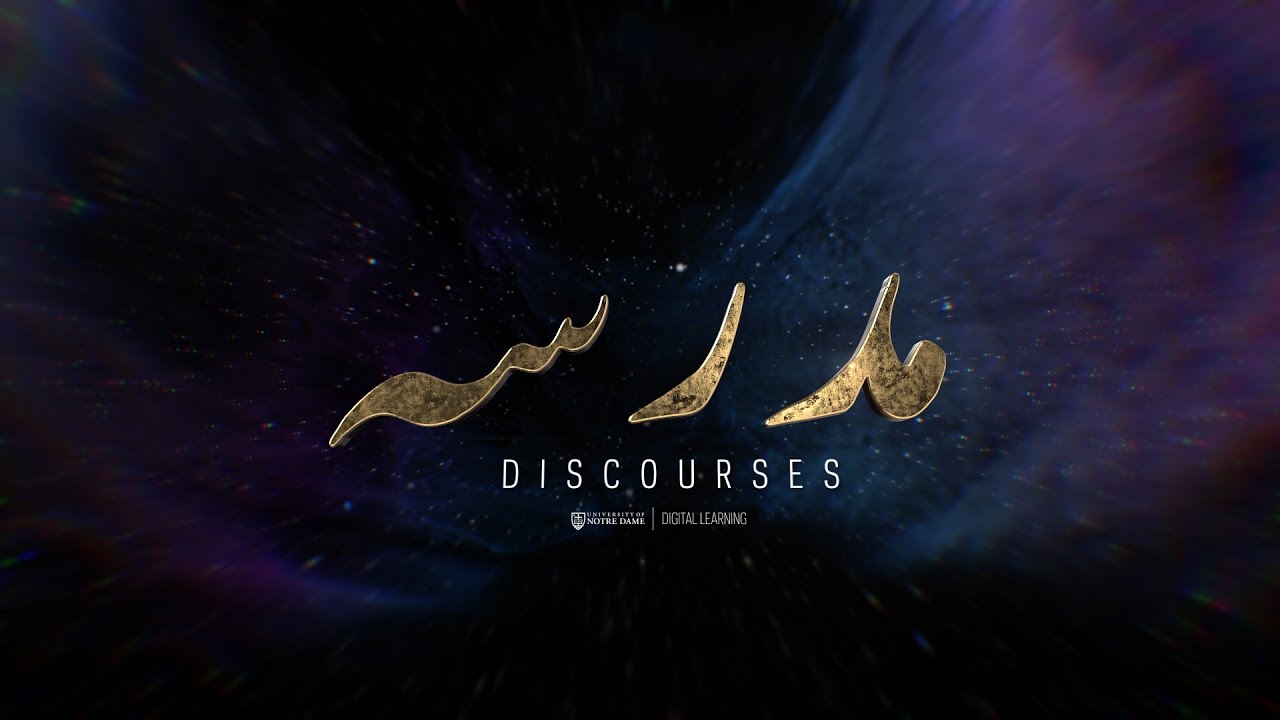This image appears to be an advertisement set against a mesmerizing, galaxy-themed background. In the center, there is a prominent white text that reads "Discourses" followed by an indistinct word and then "Learning" below it. Adjacent to the word "Learning," there is a white icon accompanied by some smaller, blurry text that's difficult to decipher. Above this central text are gold, abstract characters with a pattern that resembles black dirt or shadows. The intricate background features a navy to black gradient interspersed with purple, blue, and silver galaxy clouds, sprinkled with white stars. The whole design exudes a warp drive-like, slightly blurry yet surreal appearance, maintaining relatively clear image quality.